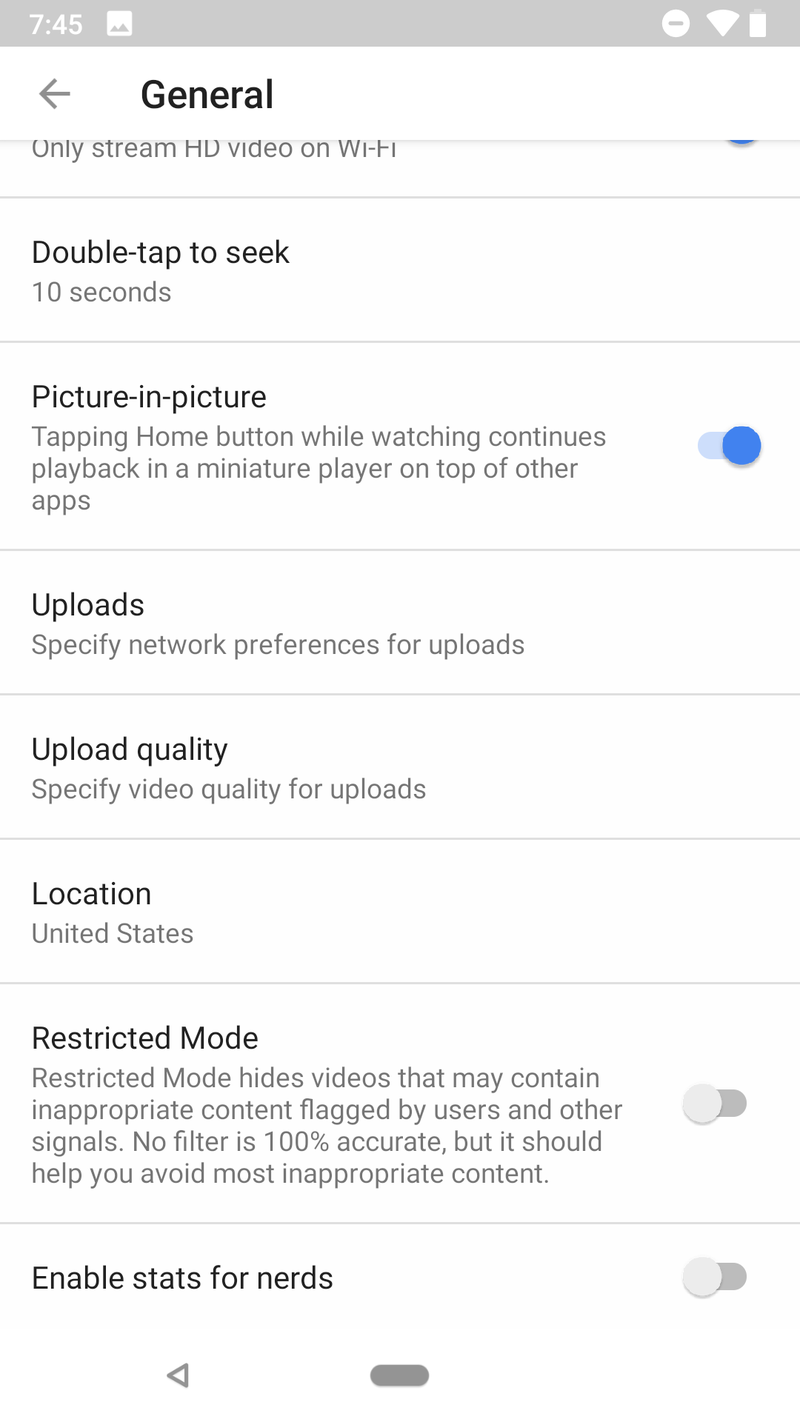This image is a screenshot from a website on a mobile device. At the very top, there is a light gray status bar. On the left side of this status bar, the time is displayed as 7:45. The right side of the status bar shows status icons: a circle with a minus sign inside (possibly indicating a Do Not Disturb mode), a Wi-Fi symbol, and a battery indicator.

Below the status bar, the page transitions into a predominantly white background. At the top left corner of this section, there is a gray back arrow. Adjacent to the arrow, black text reads "General" with a capital "G." 

The content appears to be settings related to media streaming and uploads. However, part of the text is cut off and only partially visible: "only stream HD video on Wi-Fi" is indicated as not selected. Below this is detailed as "Double-tap to seek 10 seconds" with "Picture-in-picture" option, which is selected.

Further down, settings related to uploads are listed:
- "Specifies network preferences for uploads"
- "Upload quality: Specify video quality for uploads"
- "Location: United States"
- "Restricted Mode" is noted as not selected
- "Enable stats for nerds," which is also not selected

At the bottom of the screen, a small triangle pointing left and an oval-shaped button, both in gray, are visible.